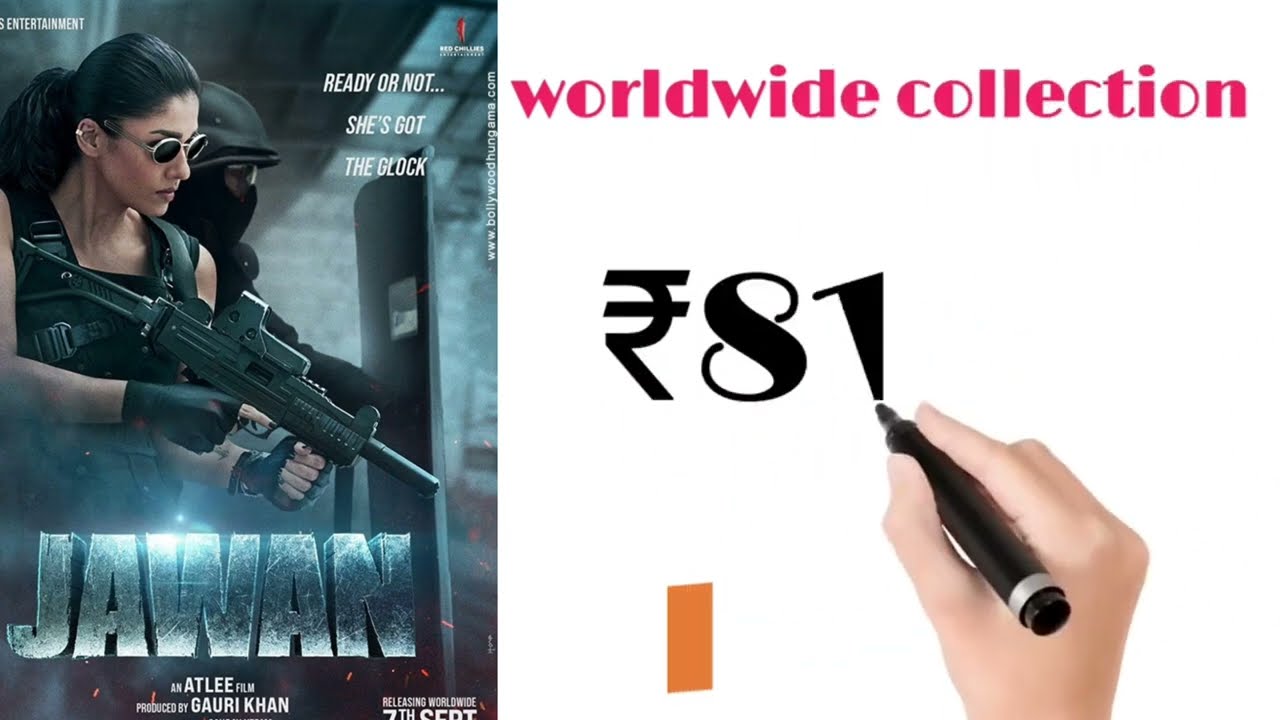The image is divided into two distinct sections. On the right side, a pure white background hosts the text "Worldwide Collection" in bold red print. Below this, there is the number "81" being written by a human hand holding a black marker, with what appears to be an unfamiliar currency symbol. A faint orange slash is visible to the left of the hand. Extending out from the bottom edge of the image, the hand is depicted to mimic the act of writing.

The left side of the image features a dramatic movie poster for a Bollywood film titled "Jawan." Central to the poster is a formidable woman with dark brunette hair slicked back into a ponytail, wearing dark gold ribbed sunglasses and a gold ear cuff. Dressed in a black bulletproof vest and tactical gloves, she wields a machine gun or high-powered automatic weapon. Positioned behind her is a man clad in a military-style helmet, face covering, and safety glasses, also holding a weapon. Additional text on the poster includes the film's title "Jawan" in a three-dimensional style, the names of the actors, and credits indicating the film is produced by Gauri Khan and directed by Atlee. The movie is set to release worldwide on September 7th, with the tagline "Ready or not, she's got the clock." The website BollywoodHungama.com is provided for further information.